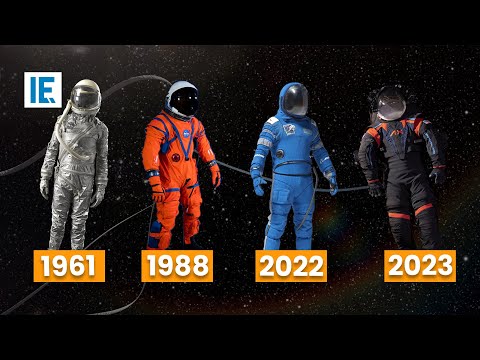The image is a poster showcasing four astronaut suits from different years against a black space backdrop adorned with white dots representing stars. In the top left corner, a white box with the blue capital letters "IE" is visible. The astronauts stand from left to right, each with a tube or string extending from their back and helmets connected by tubes to their loose-fitting, full-body suits, which obscure their feet. 

From left to right:

1. The first astronaut dons a shiny silver-gray suit with a matching silver helmet, labeled "1961" in orange text with cream-colored numbers.
2. The second astronaut wears a vivid orange suit accented with blue details and a white helmet, marked "1988."
3. The third astronaut is clad in a blue suit with white and gray accents, complete with a matching blue helmet, and the label underneath reads "2022."
4. The last astronaut sports a sleek black suit with red lines on the shoulders and thighs, along with a black helmet, labeled "2023."

A subtle silver stripe runs across the background, adding to the overall futuristic and outer space theme of the poster.